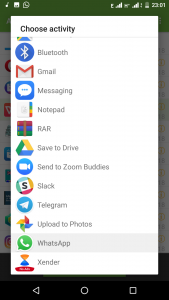The image displays a web page dedicated to selecting various activities, aptly named "Choose Activity." At the top, the text "Choose Activity" is prominently featured in black letters. 

Below this header is a series of icons accompanied by corresponding text descriptions, each representing different activities that users can choose from:

1. **Bluetooth**: A blue circle containing the Bluetooth symbol, with the word "Bluetooth" written next to it.
2. **Gmail**: The Gmail symbol, identifiable as a stylized, red-letter "M."
3. **Messaging**: Represented by a blue box featuring three white dots.
4. **Notepad**: A multicolored notepad icon, with the word "Notepad" next to it.
5. **RAR**: An icon depicting a stack of books with the text "RAR" beside it.
6. **Save to Drive**: Google's Drive triangle in green, yellow, and blue, labeled "Save to Drive."
7. **Send to Zoom Buddies**: A camera icon inside a blue circle, labeled "Send to Zoom Buddies."
8. **Slack**: A multicolored circle with an "S" in the center, representing Slack.
9. **Telegram**: A blue circle containing a paper airplane symbol, representing Telegram.
10. **Upload to Photos**: A multicolored windmill icon accompanied by the text "Upload to Photos."
11. **WhatsApp**: A green icon featuring a phone symbol, labeled "WhatsApp."
12. **Zender**: A yellow and blue hourglass icon, labeled "Zender."

Each icon and description is clearly structured, making it easy for users to identify and choose their desired activity.